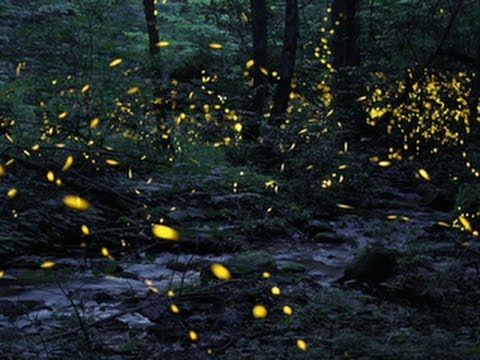The image illustrates a mesmerizing nighttime forest scene, where a dark, almost blackish-gray stream or brook, frothy with white foam, snakes through the landscape. Black trees with green leaves frame the scene, and boulders and rocks punctuate the flowing water. The forest is dimly lit, likely by minimal moonlight, creating a serene, shadowy backdrop. Fireflies, emitting a delicate yellow glow, dominate the scene, swirling in intricate patterns mainly in the center and some resting atop the trees. Their luminescence provides a stark contrast to the dark surroundings, casting a constellation of sparkling lights that infuse the forest with an ethereal charm. Dotted with green plants and sticks, this tranquil nighttime image captures the enchanting dance of fireflies in an outdoor forest setting.